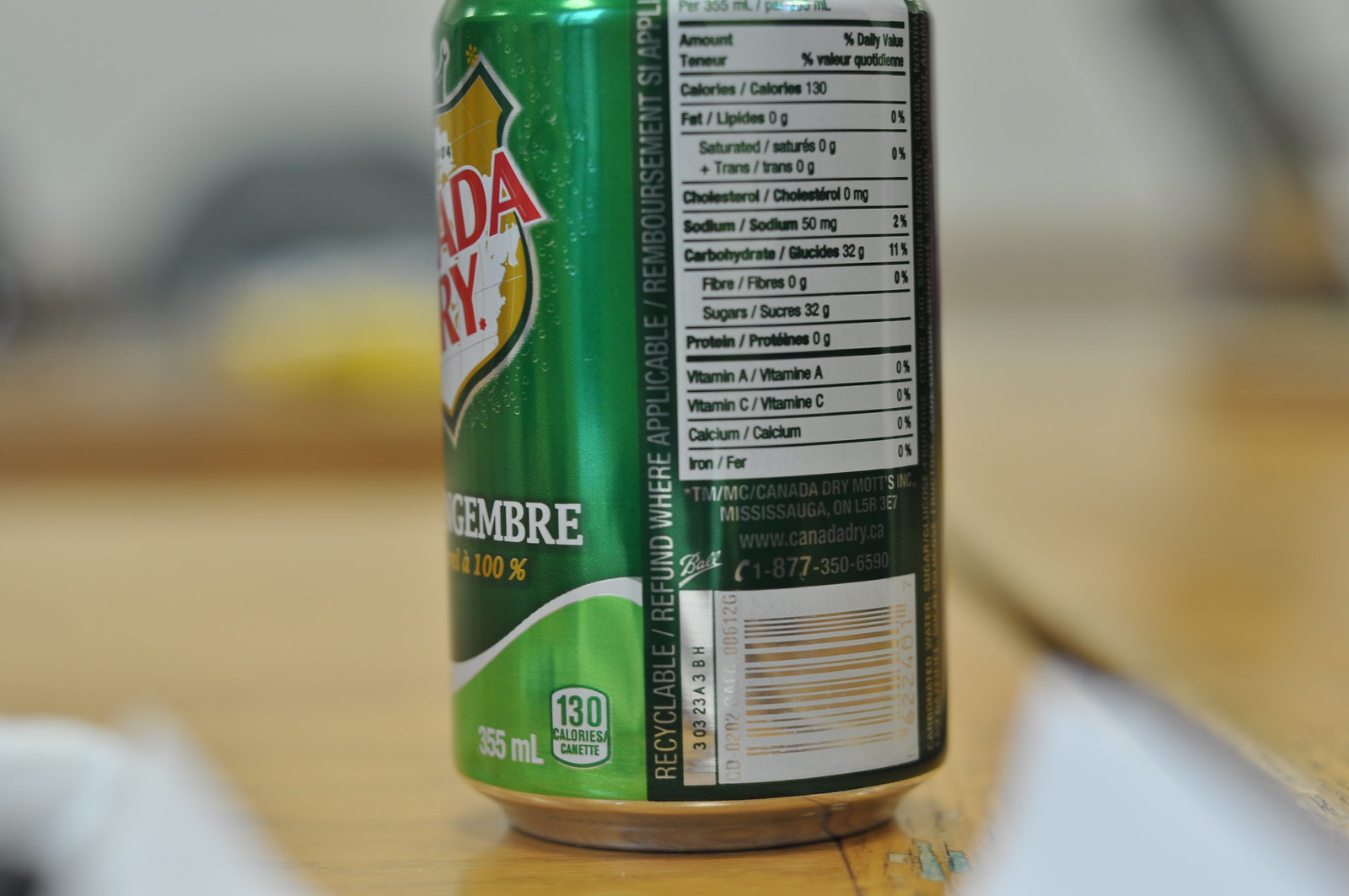This is a close-up photograph of a green can of Canada Dry, positioned atop a light wood grain surface with a blurred background. The can features a prominent dark green color with accents of light green, white, and silver. Visible are the back half of the can, including an ingredients list, nutritional facts—detailing 130 calories per 355 milliliters—and a white and silver barcode. Alongside this section runs a vertical line of silver text that reads "recyclable refund where applicable." To the left of this text is part of a gold and white logo, resembling a sheriff's badge, with additional white detailing and red text above it. The image captures intricate design elements, including a small white stripe in the middle of the can and the prominent logo partial on the front, emphasizing the meticulous branding of the Canada Dry beverage.